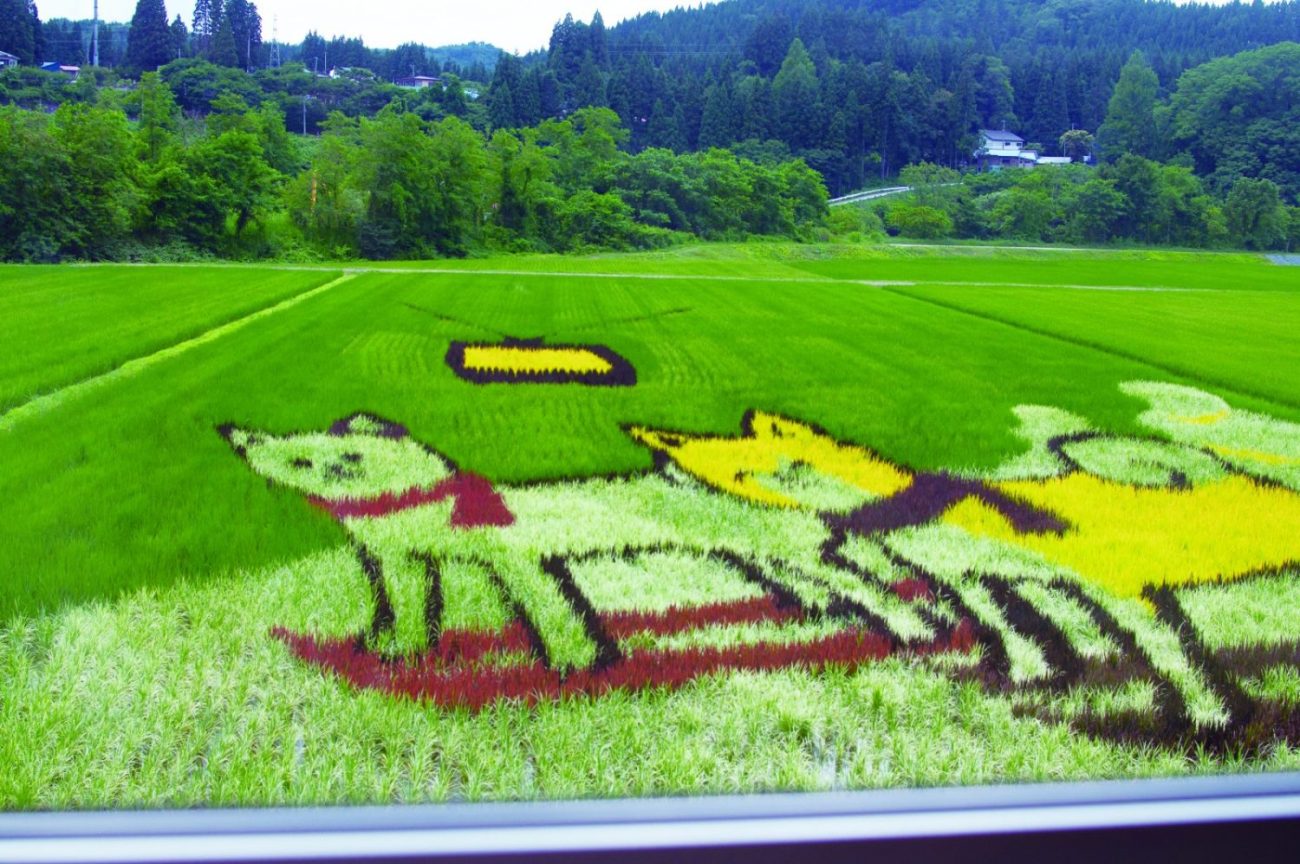The image is a vivid color photograph of a lush green field, flanked by bright green trees and hills in the background, forming a vivid natural setting. The field is dominated by a central painted section, creatively transformed into stylized images of two animals. The animal on the left is a lightly green dog with black outlines, wearing a maroon scarf, and is positioned on red patches of grass. The dog on the right is yellow, also outlined in black, wearing a black scarf, and is standing on black patches of grass. Both animals, resembling either dogs or cats, have small ears and are front-facing, looking slightly to their left. Above them, there is a prominent black and yellow square, possibly resembling a television set with antennae. The field appears well-maintained, and the vivid colors of the animals against the bright green surroundings make for a striking and playful image set in this open, picturesque space.